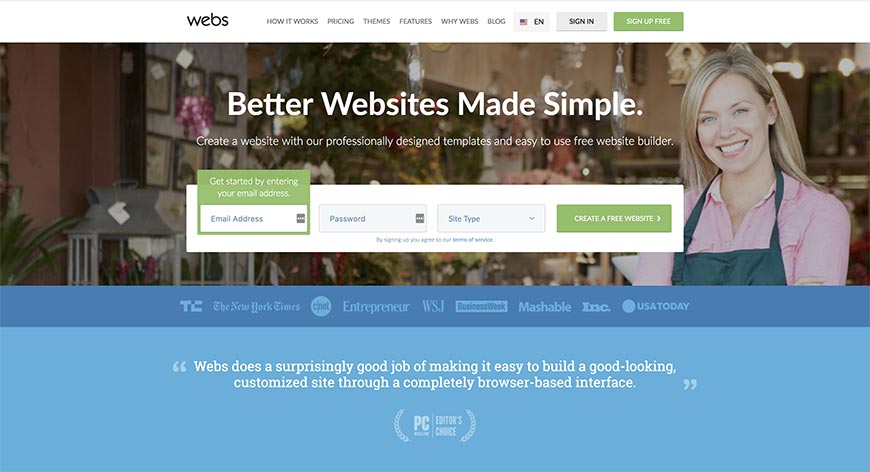This image captures a screenshot of a website's homepage. At the top, a banner spans the width of the page, featuring navigation menu options. The menu includes items such as "How It Works," "Pricing," "Themes," "Features," "Why Webs," "Blog," and a language selection button that defaults to English. Additionally, there are sign-in and green sign-up buttons with white text.

The central portion of the webpage is dominated by a large rectangular section. The upper part of this section displays an image of a woman inside a retail setting. Overlaying the image is the tagline: "Better websites made simple. Create a website with our professionally designed templates and easy-to-use free website builder."

Below the image, a form is provided for users to get started. It includes fields for entering an email address, password, selecting a site type from a dropdown menu, and a button to create a free website.

Directly beneath the form, there is a dark blue bar showcasing the logos of various prominent publications, such as The New York Times, CNET, Entrepreneur, The Wall Street Journal, Businessweek, Mashable, Inc., and USA Today, indicating endorsements or features about the website.

At the bottom of this section is a highlighted quote stating: "Webs does a surprisingly good job of making it easy to build a good-looking customized site through a completely browser-based interface." This testimonial is credited to PC Magazine's Editor's Choice.